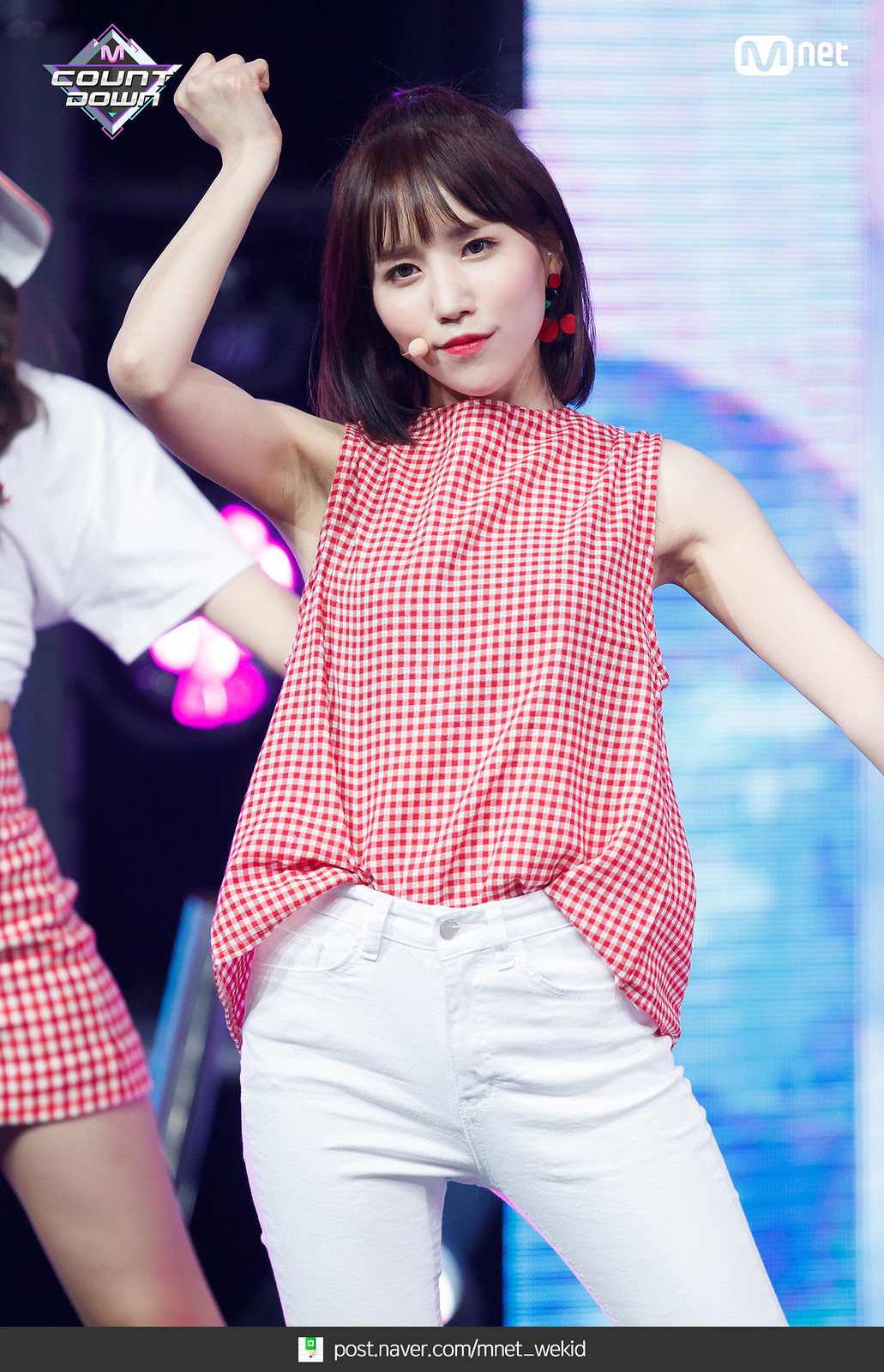The photograph captures an Asian woman performing on stage, likely in an event organized by MNET, as indicated by a watermark in white text at the top right corner and a diamond logo with "Countdown" in white text on the top left corner. At the bottom, a gray banner displays the text "post.naver.com/MNET_WeKid." The performer, who has short shoulder-length black hair, is energetically posing with her right arm raised in a fist. She is wearing white jean pants with a front button, along with a sleeveless black, red, and white tank top that features a red and white checkered pattern, reminiscent of a picnic blanket. She has cherry earrings that dangle from her ears, and her face is adorned with red lipstick. Attached to her face is a pink microphone, indicating that she is mid-performance. To the left, there's another woman partially visible, showing only her leg, which is clad in a skirt made from the same red and white checkered fabric as the performer's shirt.